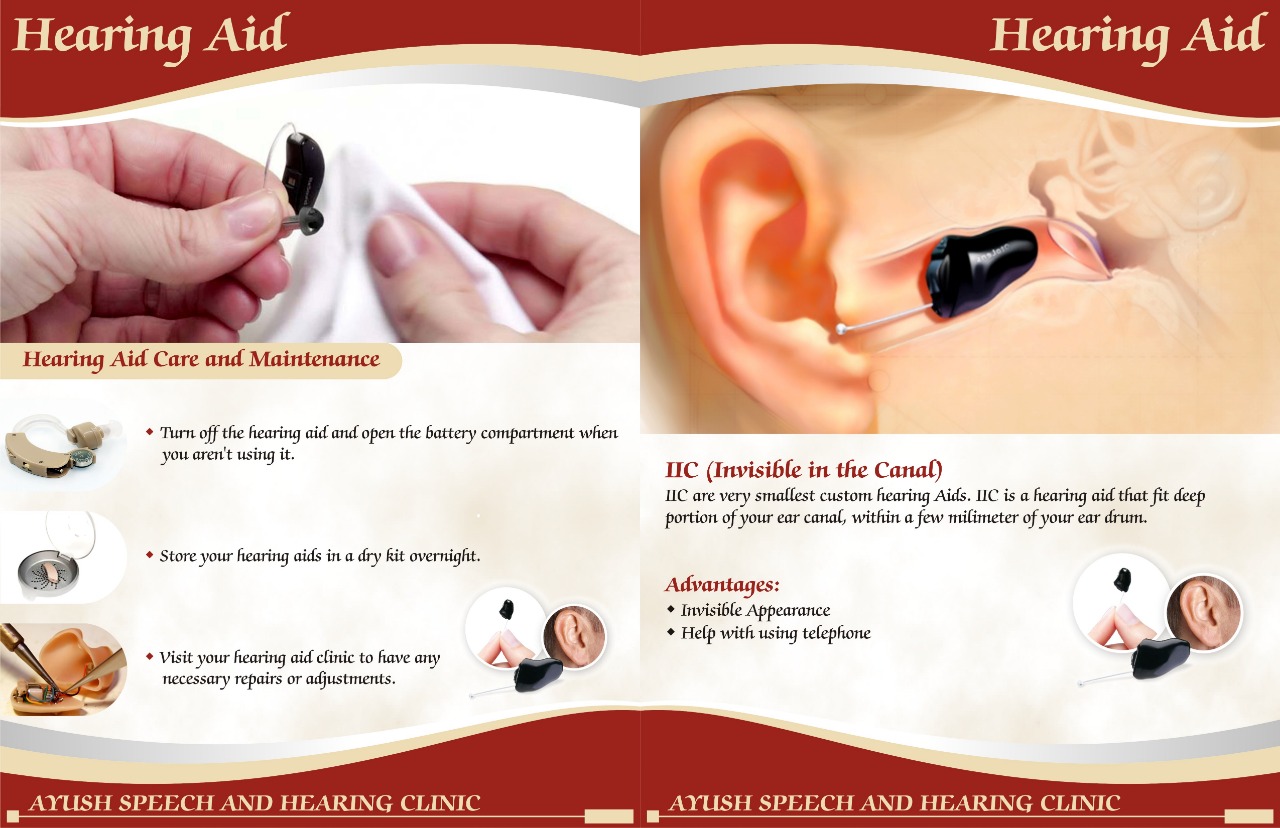The image is a detailed digital brochure, split into two pages side by side, focusing on hearing aid care and maintenance. Dominated by a red border with wave patterns at the top and bottom, the brochure prominently features the words "Hearing Aid" in yellow on both the left and right corners at the top. Below, in a yellow box framed by red letters, is the heading "Hearing Aid Care and Maintenance." The right side of the brochure shows a hand delicately holding a black hearing aid and a white handkerchief, alongside diagrams and illustrations of the hearing aid’s placement in the ear. This section emphasizes the proper insertion of the hearing aid into the ear canal, featuring a realistic ear and an interior drawing to show the fit. A bullet point list provides maintenance instructions and the advantages of using the hearing aid, set against a white background. The bottom includes the text "IU Speech and Hearing Clinic" on both sides. Further illustrations depict various types and sizes of hearing aids, with descriptive text clarifying their use and care.